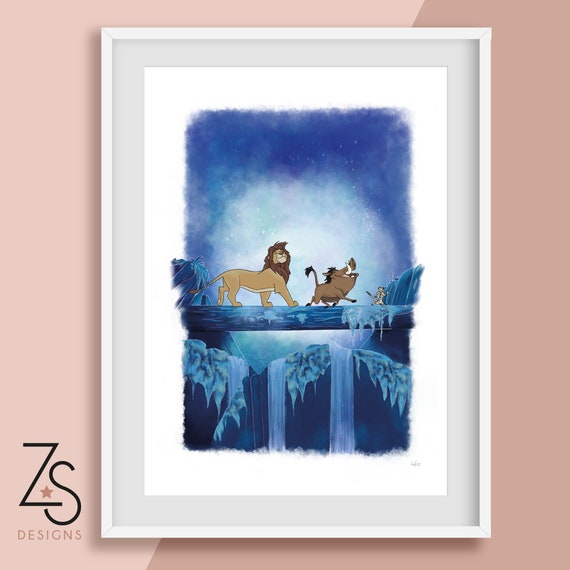The image depicts a framed painting or screen grab from the animated Disney movie, The Lion King. The scene features Simba, a tan lion with a lighter underbelly and a brown mane, walking alongside Pumbaa, a brown warthog with black hair on top of his head and white curved tusks, and Timon, a meerkat that is tan on the back and white on the front. They are crossing a river by walking on a log, which takes on a blue hue, against a backdrop of a blue sky with hints of white and a full moon-like cloud. The vibrant and brightly lit image is very clear and mounted on a wall that appears to be a combination of tan, peach, and light purple. The white frame contrasts with the colored walls, and in the lower left corner, the text "ZS Designs" is visible, suggesting an artist or brand signature.